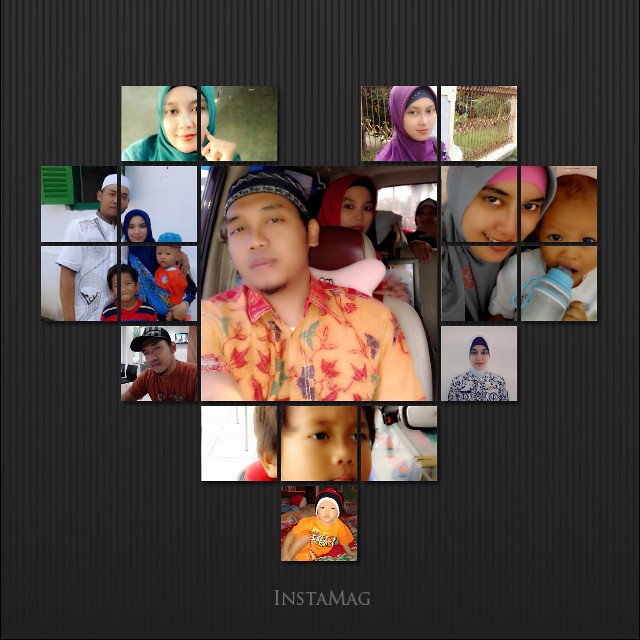The image is a detailed collage of family pictures set against a black background with darker black vertical stripes, somewhat resembling gray and black tubes. In the center of the collage, there's a prominent square photo of a man adorned in a red and orange button-up shirt and wearing a black cap or bandana. He appears to be seated in the front passenger seat of a vehicle, with several people visible in the seats behind him, suggesting he might be in some type of van or bus.

Surrounding this central image, the collage is meticulously divided into quadrants, each delineated by vertical and horizontal black lines. These quadrants feature various snapshots of the family: a woman wearing differently colored head coverings—green, purple, gray, and dark blue—, a baby drinking from a plastic bottle with a blue top, and another baby at the bottom of the collage, dressed in an orange outfit and a red, black, and white tuque. There is also a family photograph including the man, the woman, and two children, neatly bisected by prominent black lines. This thoughtfully assembled collage captures moments and members of the family, providing a warm, detailed visual narrative. A gray-font watermark reading "Instamag" is positioned at the bottom of the image.